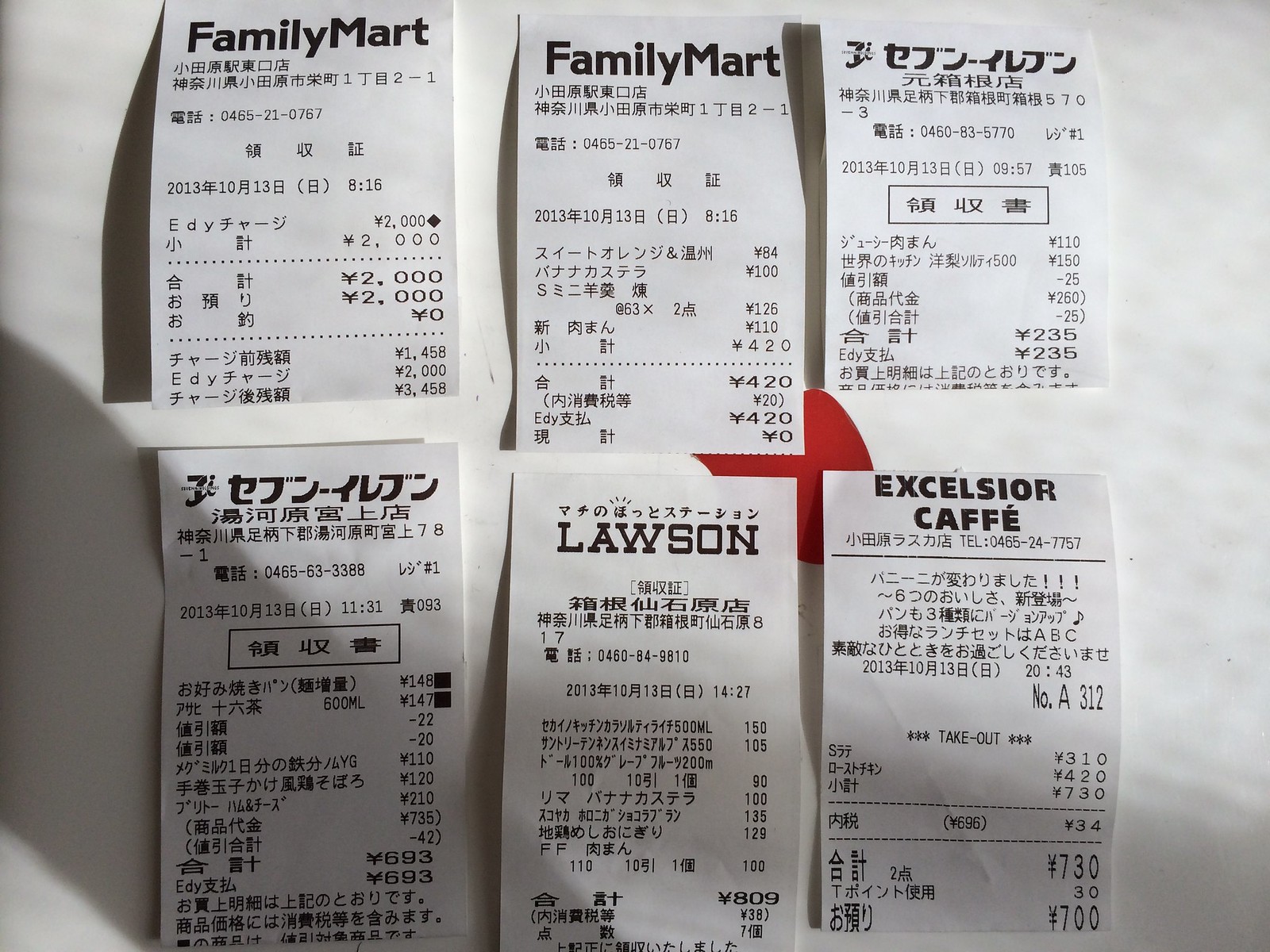The image is a color photograph of six till receipts from various Japanese commercial establishments, meticulously arranged in two rows of three on a predominantly white surface. The upper row consists of two receipts from Family Mart on the left and middle, each containing dense traditional Japanese characters alongside numbers indicating purchase details, times, dates, and balances—specifically 2,000 yen and 420 yen. The top right receipt, though largely in Japanese, does not specify the establishment in the captions provided.

The bottom row features a mix of receipts from distinctive places. The middle receipt, prominently labeled "LAWSON" in English, also contains detailed Japanese text and a balance of 809 yen. The bottom right receipt is from "Excelsior Café," notably misspelled with two Fs as "EXCELLSIA CAFE," showing Japanese characters and an itemized list culminating in a balance of 730 yen. The bottom left and middle receipts within this row represent another unidentified Japanese store but include comprehensive numerical data and Japanese script, with respective balances of 235 yen and 693 yen.

Interestingly, the receipts are not lying flat; they retain a slight curvature from being just unrolled. The setting appears to feature a marble-like white surface, interrupted by a small, undeciphered red geometric shape underneath the receipts, vaguely reminiscent of the Japanese flag. The bottom left-hand corner features a shadow across the corner receipts, possibly cast by the photographer's arm or the camera flash.